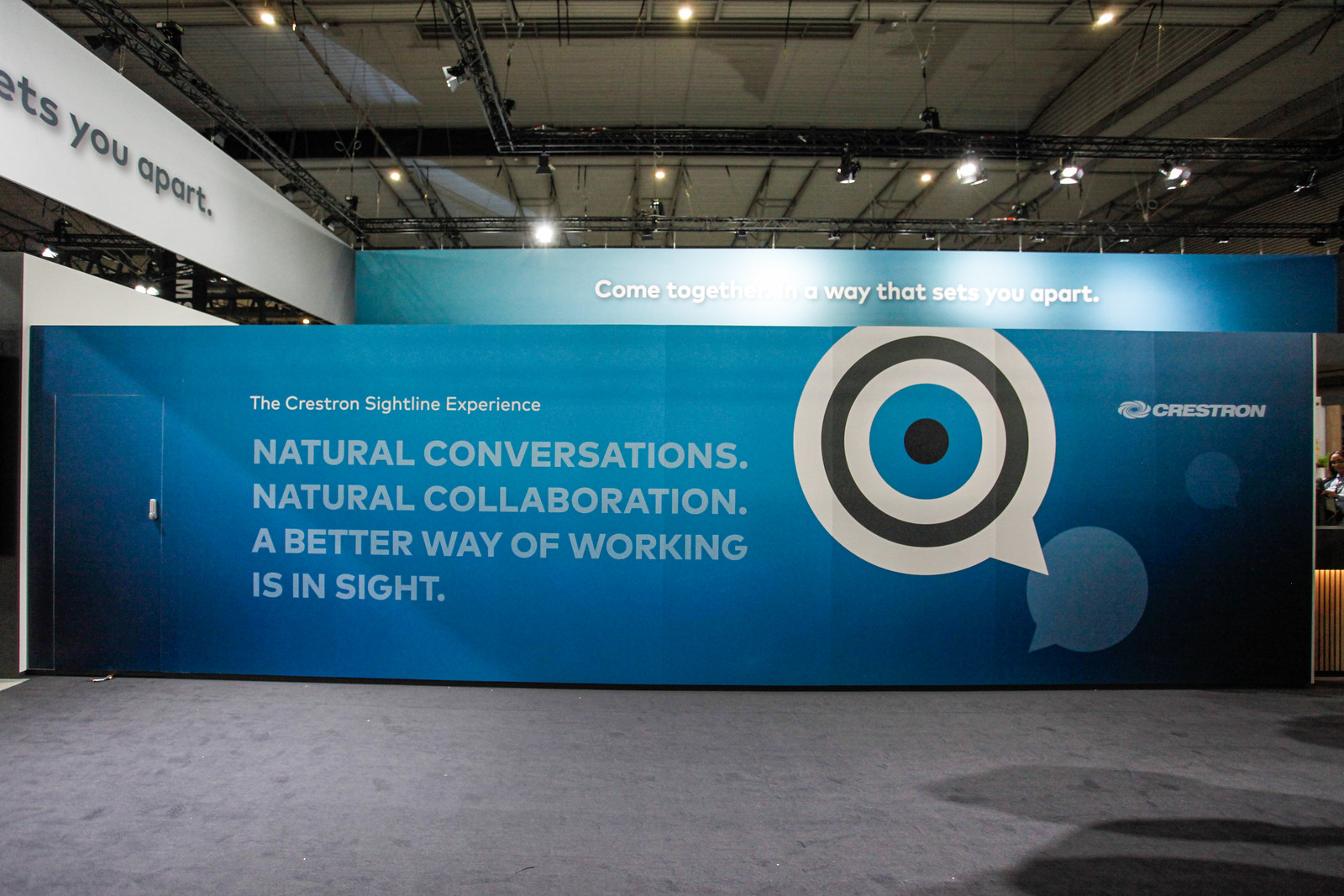The image captures a large advertisement on a prominent wall within what appears to be a convention or warehouse venue. The advertisement prominently features the word "Creston" along with its logo on the right side, both set against a blue-themed background that fades from dark to light blue. At the top, the text reads, "Come together in a way that sets you apart." To the left of the logo, a large speech bubble forms the shape of a human eye with a blue iris, containing the slogan, "The Creston Sightline Experience. Natural conversations, natural collaboration, a better way of working is in sight." The wall includes architectural elements like a door, and the overall setup indicates a vision of advanced, seamless collaboration. The background reveals elements of the building's interior, including ceiling structures.